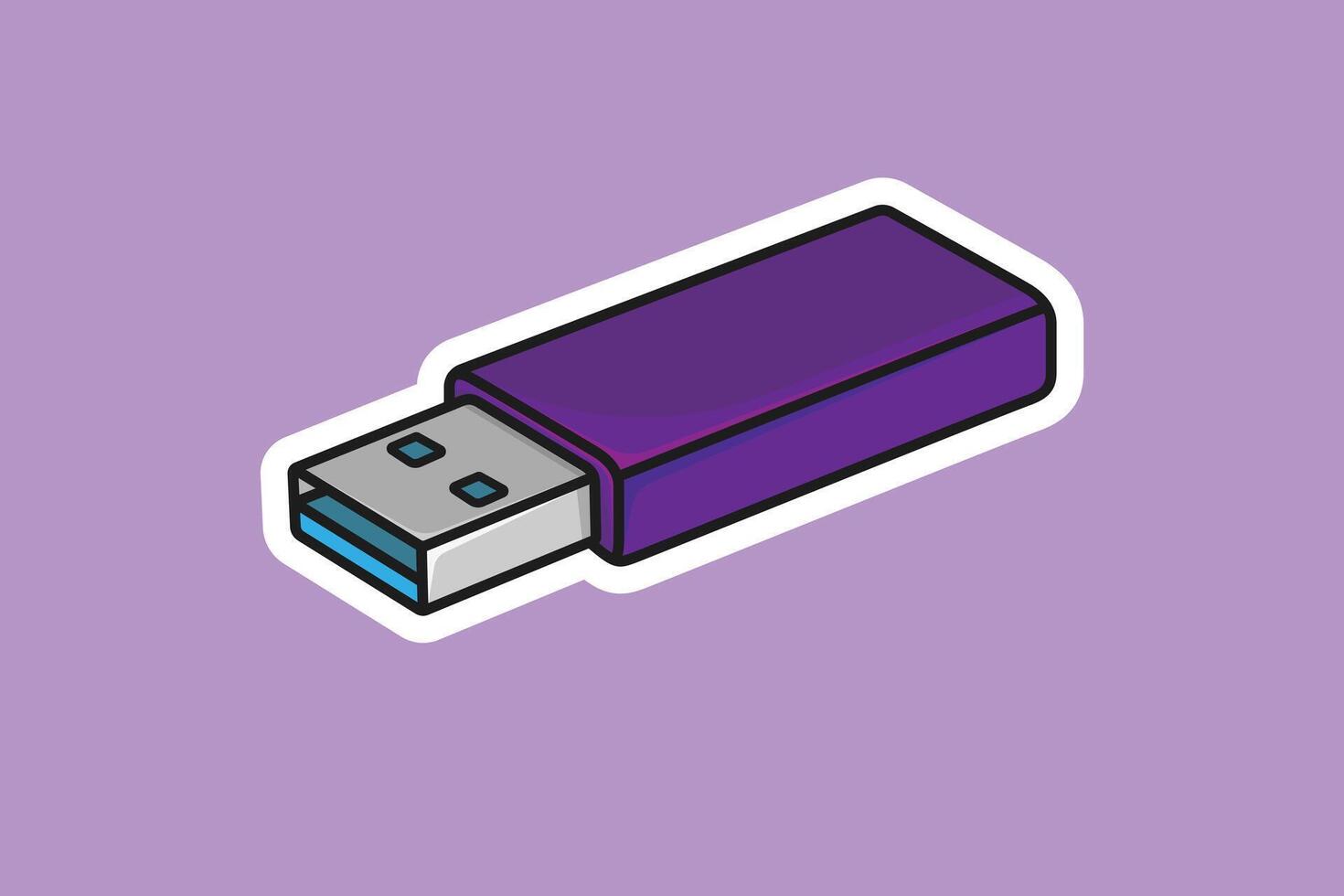The image is a digital, animated illustration of a USB-A stick, which is a type of jump drive used to store data. The drive is a small rectangular shape, primarily dark purple with a black outline and further highlighted by a thick white border, giving it a somewhat circular appearance overall. The part of the USB stick that is inserted into the computer is grayish silver and features two teal squares in its middle, outlined in black. This section also shows the inside mouth part with a matching teal color, transitioning to more of a blue hue below it. The USB stick is set against a lavender background, which accentuates its purpleness and clean, proportional design. The image is highly symmetrical with subtle gradients, making the structure appear slightly 3D and blocky, while maintaining an overall crisp and neat visual quality.